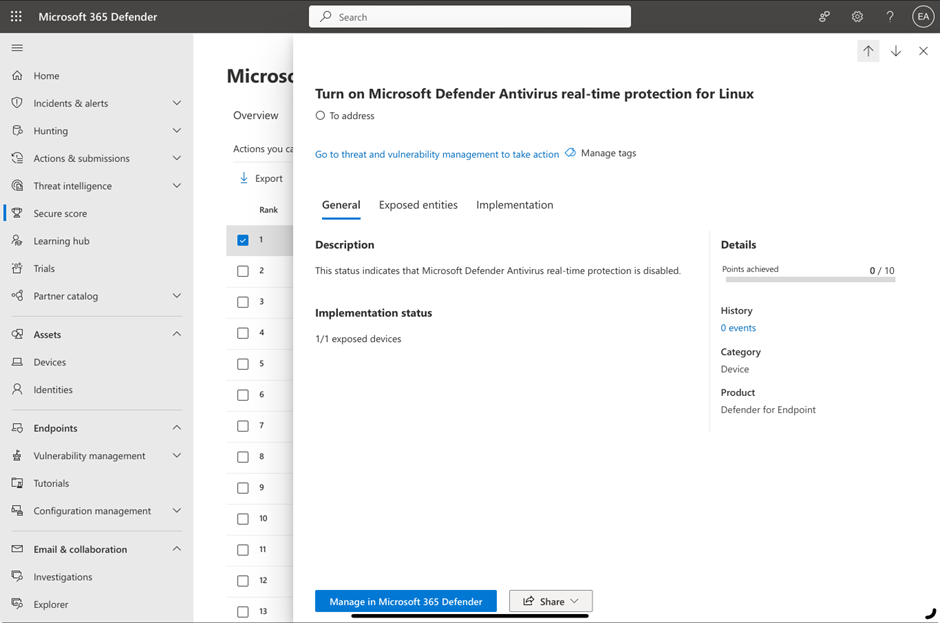Caption:

In this screenshot of the Microsoft 365 Defender interface, specifically tailored for Linux, we see a detailed context menu. The left-hand sidebar is cluttered with overlapping options, including Home, Incidents and Alerts, Hunting, Actions and Submissions, Threat Intelligence, Secure Score, Learning Hub, Trials, Partner Catalog, Assets, Devices, Identities, Endpoints, Vulnerability Management, Tutorials, Configuration Management, Email and Collaboration, Investigations, and Explore.

At the forefront is an open menu with a search bar above. A prompt reads, "Turn on Microsoft Antivirus Real-Time Protection for Linux," with a highlighted action circle labeled "To address." This navigates users to Threat and Vulnerability Management for action and tag management.

The currently highlighted tab, "General," is underlined. Its detailed contents indicate that Microsoft Defender Antivirus Real-Time Protection is disabled. It provides a status overview, showing "One exposed device," "Zero of ten points achieved" under Details, and "Zero events" in History. The category is listed as "Device," and the product as "Defender for Endpoint."

Additional tabs next to "General" include Exposed Entities and Implementation. At the page’s bottom middle, there's a blue link for "Manage in Microsoft Windows, Microsoft 365 Defender" and a Share button with an adjacent context menu. In the background, there is a partly visible section labeled "Overview" among other indistinct options.

The interface reflects the somewhat incongruous adaptation of Microsoft Defender for Linux, demonstrating a comprehensive yet busy layout.